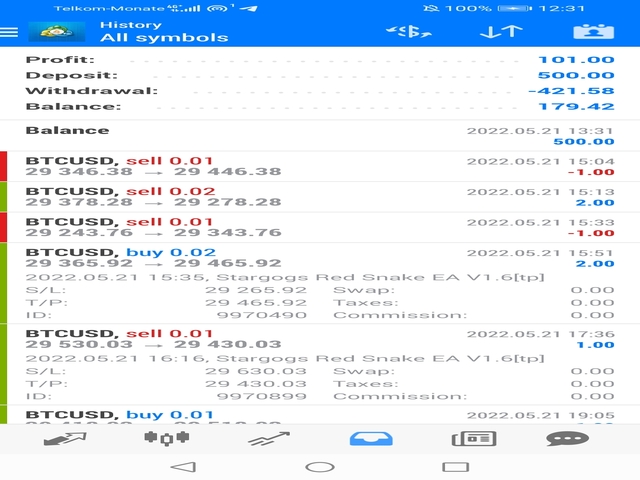A pixelated and slightly blurry screen capture of a smartphone displaying a financial trading app. The top of the image features a bright blue banner with three horizontal white lines on the left, indicating a menu button. To the right of this is a money icon followed by "history all symbols." Above this, the network name "Takam Manate" is displayed along with 4G connectivity status, four Wi-Fi bars, a letter M, and an airplane-like up arrow. On the far right, it shows the time as 12:31, 100% battery, an up arrow, and a down arrow, as well as a white rectangle with a human icon resembling a Rolodex card.

Beneath the banner, the main section of the screen is filled with a white background listing various financial headings such as profit, deposit, withdrawal, and balance. There are multiple rows of financial data marked with alternating red and green bars on the left, indicating the fluctuations in stock or investment values, particularly BTQs and QsD. Sell numbers are displayed in red while buy numbers are shown in blue.

On the right-hand side of each row are the dates and the related financial figures, detailing both expenditures and earnings. 

At the bottom, in a slightly off-white banner, there are various icons from left to right: an up and down arrow, a settings gears icon, an unfamiliar icon with a zigzag line and two lines beneath it, a blue and white inbox, a square with paragraph lines, a speech bubble with three dashes. At the very bottom against a white background are a gray left-pointing arrow, a circle in the center, and a rectangle on the far right.